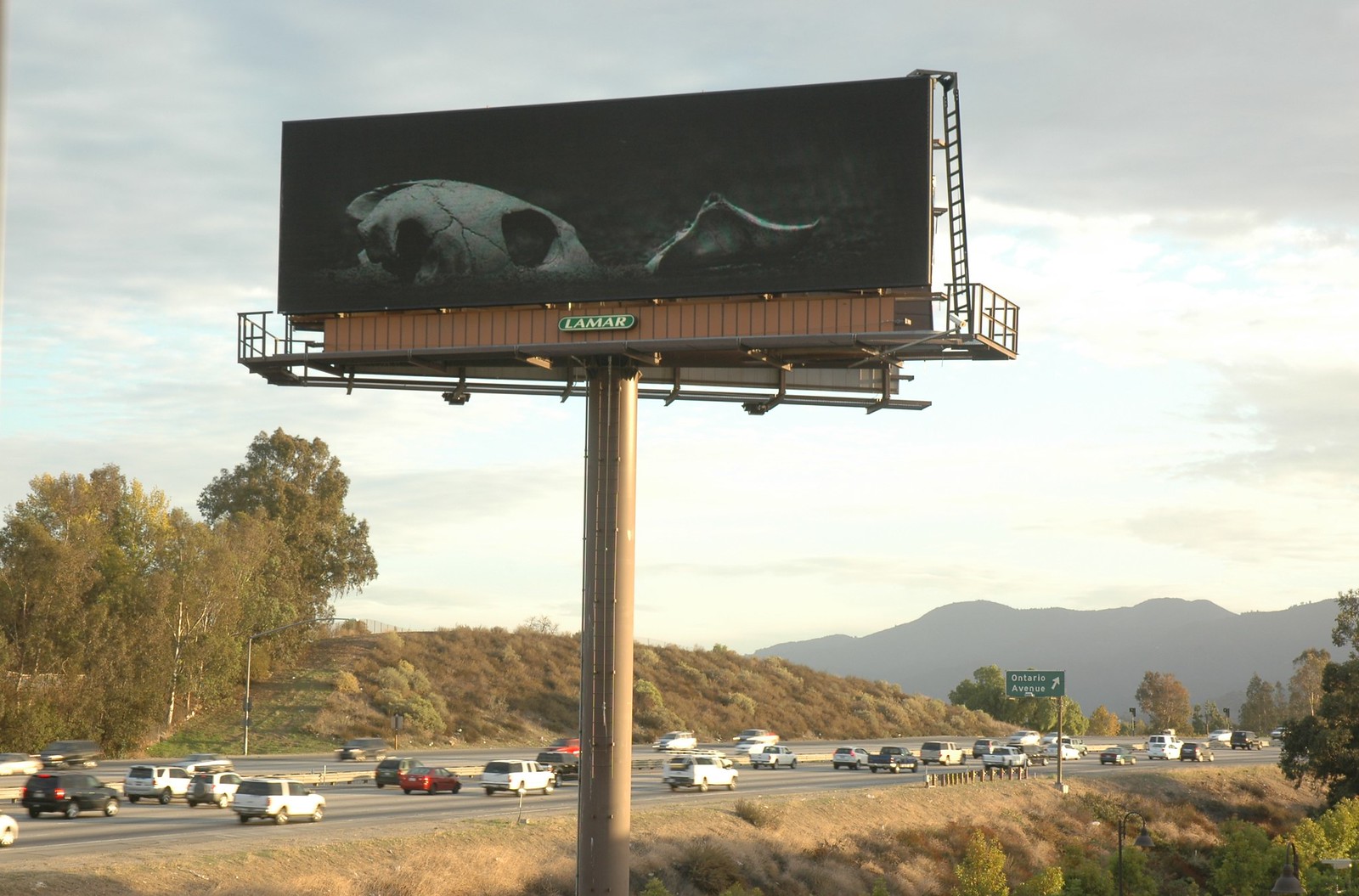This photograph captures a towering billboard mounted on a robust column, soaring multiple stories above a bustling multi-lane freeway. The billboard itself is stark black, featuring a striking image of an animal skull. Vehicles of various types speed along the freeway in both directions, which occupies the lower portion of the image. In the background, rolling hills stretch across the horizon, dotted with patches of brown vegetation. A green highway sign indicating "Ontario Avenue" suggests the presence of an off-ramp. The scene is framed by dry, brown vegetation in the foreground and background hills, adding to the dramatic and somewhat desolate atmosphere of the landscape.